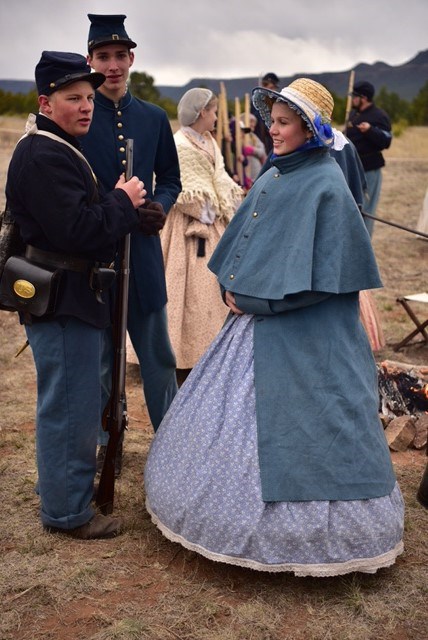This image captures a detailed scene from a Civil War reenactment, vividly brought to life by a professional photographer. The main focus is on three individuals in traditional attire, standing in a grassy, dirt field with hills and cloudy skies in the background. On the left, a tall gentleman is dressed in a dark blue jacket, light blue pants, and brown boots, completed with a black leather knapsack adorned with a gold symbol. He wears a dark blue hat with a gold button and holds a musket gun as he looks off into the distance. 

Next to him, another man in similar Civil War attire—a dark blue long coat with gold buttons and matching hat—stands slightly behind, gazing more directly at the camera. 

On the right, a woman stands out in a light blue dress decorated with white flowers and white lace trim. She wears a cerulean blue cape over her back and a straw sun hat with a blue ribbon. She is turned to the left with a warm smile, her dress slightly flared and extending almost to the ground. 

In the backdrop, bits and pieces of other participants dressed in period clothing, including a woman in yellow, add to the authenticity of the scene. The overall atmosphere is one of shared enjoyment and historical immersion, with everyone appearing happy and engaged in their roles.